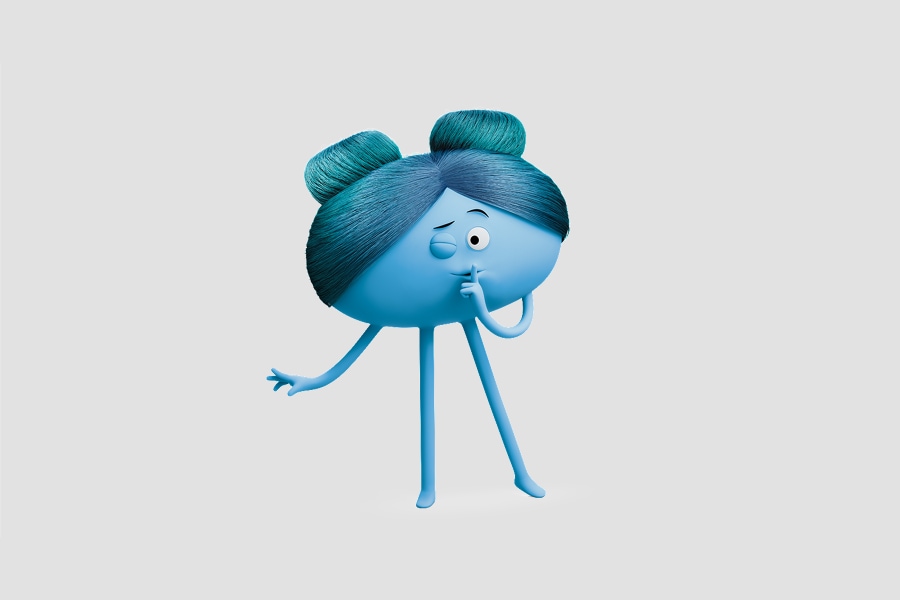An animated character from the movie "Inside Out" is depicted against a solid gray background. The character, which is shaped like a jelly bean, is light blue with straight blue hair parted in the middle, cascading to the sides, and tied into two buns at the back. Its expressive face shows one eye open with an arched eyebrow, while the other eye is winking. The character's lips are pursed, and a tiny, delicate arm extends with a finger held to the lips, suggesting silence. This character has extremely long and thin limbs, adding to its whimsical appearance.